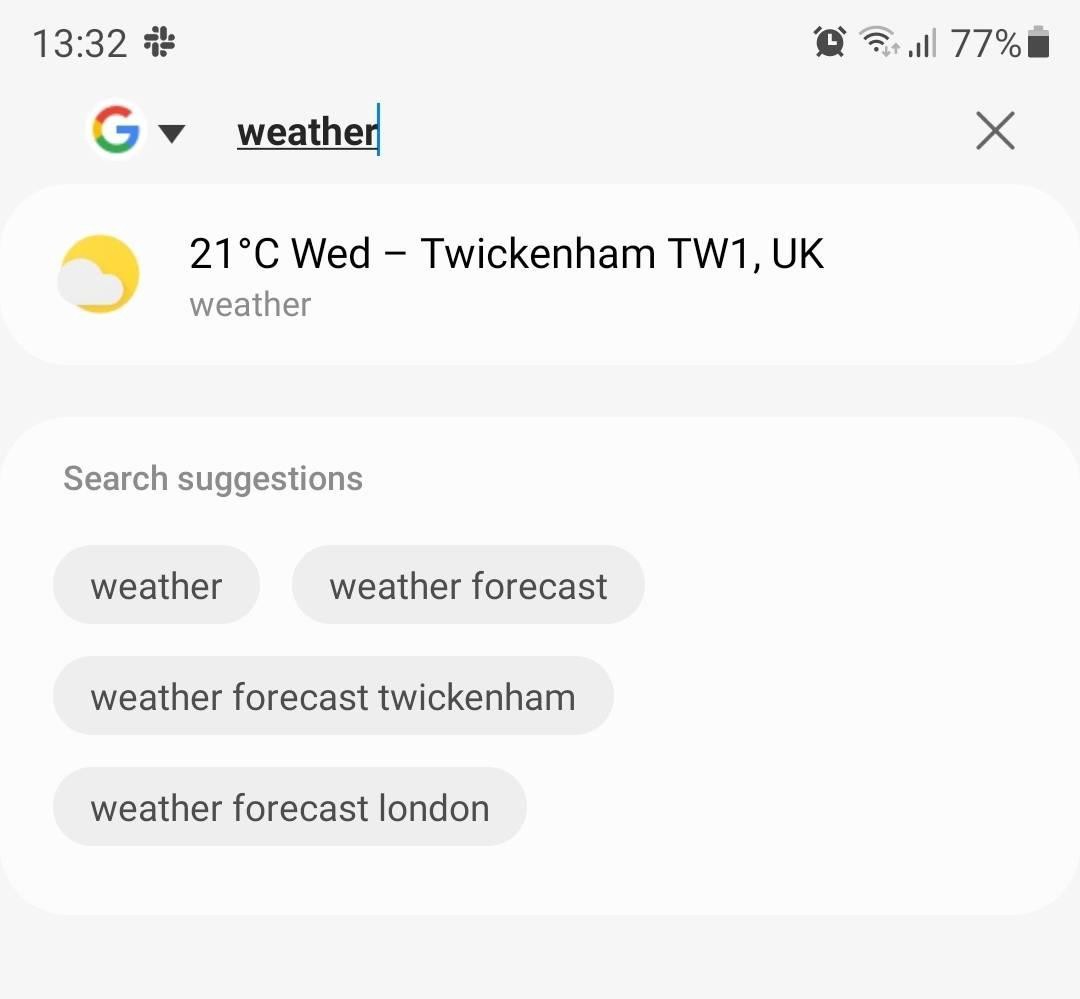Here's a cleaned-up and detailed caption for the described image:

---

The image displays a weather website interface against a gray background. At the top left, the time '13:32' is prominently shown. Next to the time, a small black flower-like icon is visible. Moving to the right, an alarm clock icon appears, followed by the Wi-Fi connection symbol. Further right, the battery level reads '77%' alongside a battery icon.

Beneath this top bar, a Google search bar is positioned. The large Google 'G' logo is to the left of the search box, which contains the query "weather." An 'X' icon to the right of the search box allows users to clear the input.

Below the search bar, there's an icon depicting a sun partially obscured by a cloud. Adjacent to this weather icon, the temperature reads '21°C.' The text beneath specifies "Wednesday Twickenham TW1 UK weather" in black and gray.

A white suggestion box is located below this weather summary. It features four clickable suggestions with small icons: 'weather,' 'weather forecast,' 'weather forecast Twickenham,' and 'weather forecast London.' Each suggestion is enclosed in a separate gray box with black text.

---

This caption thoroughly details all interface elements and their layout, providing a clear and descriptive overview of the weather website screenshot.